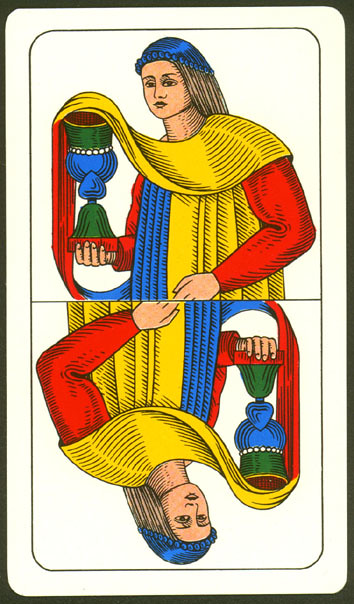This image features a unique and intricately detailed reverse design that resembles a playing card or a tarot card. The artwork is set against black outer edges which frame a central white card, trimmed with a thin black border. This gives it the appearance of a classic solitaire card, but with a creative twist.

The card is visually divided into two halves by a horizontal black line. The top half displays a meticulously illustrated image of a figure, potentially a lady or man with Caucasian features. The person has long, straight blond hair adorned with a blue headdress. They are dressed in a half-yellow, half-blue garment, with additional red long sleeves visible underneath. A vibrant yellow sash drapes gracefully over their shoulder and intersects with a red and blue section toward the bottom of the image. 

In the person’s right hand, they hold a pot or chalice, characterized by vivid colors and intricate designs. The base of the chalice is red, transitioning into a green section, then narrowing into a thin part before expanding into a blue bulbous segment adorned with a white pearly motif. The top of the chalice is green, maintaining the color scheme and design complexity.

The bottom half of the card mirrors the top half perfectly, flipped upside down. This symmetrical inversion enhances the card’s striking visual impact, making it resemble a mirrored reflection and adding a layer of mystique akin to traditional playing or tarot cards.